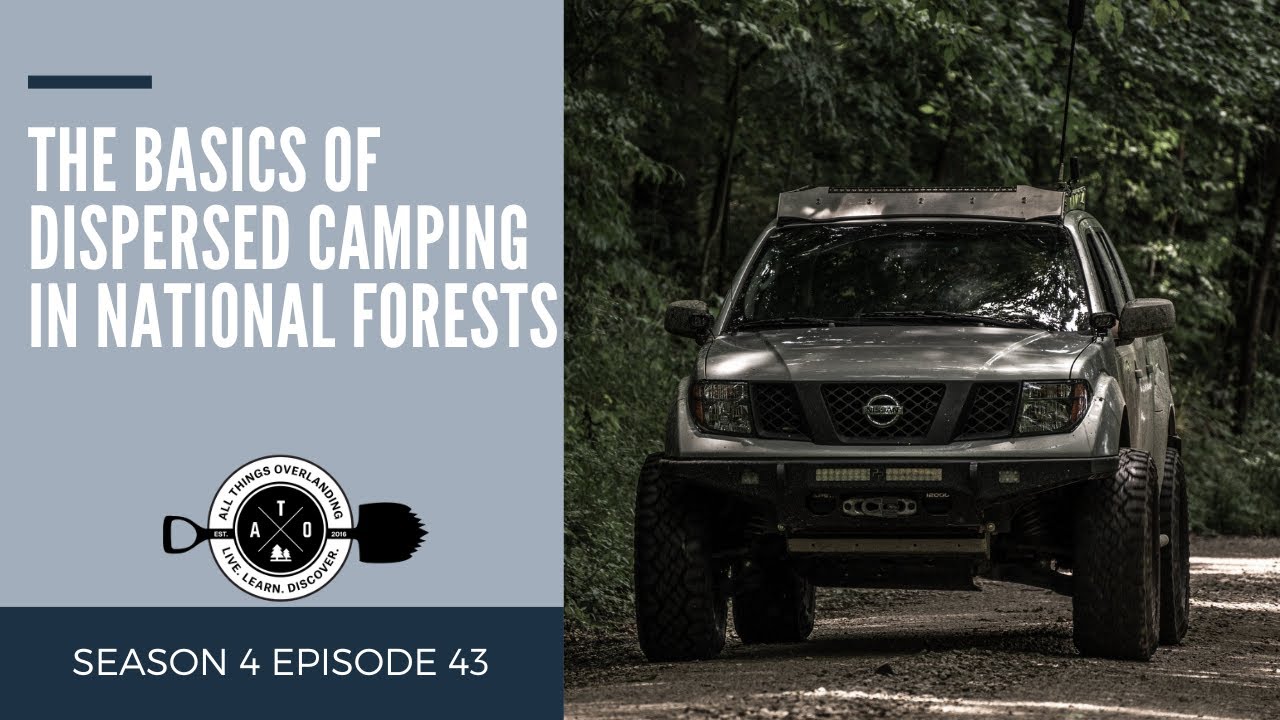This is a detailed poster advertisement related to car camping, specifically focusing on dispersed camping in national forests. The poster is oriented panoramically and divided into two key sections.

On the right side, there is a photograph of a silver four-door Nissan pickup truck positioned in the shadows of trees along a gravel road, with large wheels and a luggage rack on top. The truck is facing forward on the road, surrounded by green bushes, conveying a rugged, adventurous vibe.

On the left side, the background transitions to a mix of baby blue and navy blue areas. Prominently displayed in white text, it reads, "The Basics of Dispersed Camping in National Forests." Below this text, there is a circular logo featuring a black shovel passing through it, encircled by the phrases, "All Things Overlanding, Live, Learn, Discover," along with the acronym "A-T-O" inside a black circle with a white X. At the bottom of the left section, in additional white text on a dark blue background, it is noted as "Season 4, Episode 43," indicating that this poster is likely for a vlog or video series about overlanding and car camping.